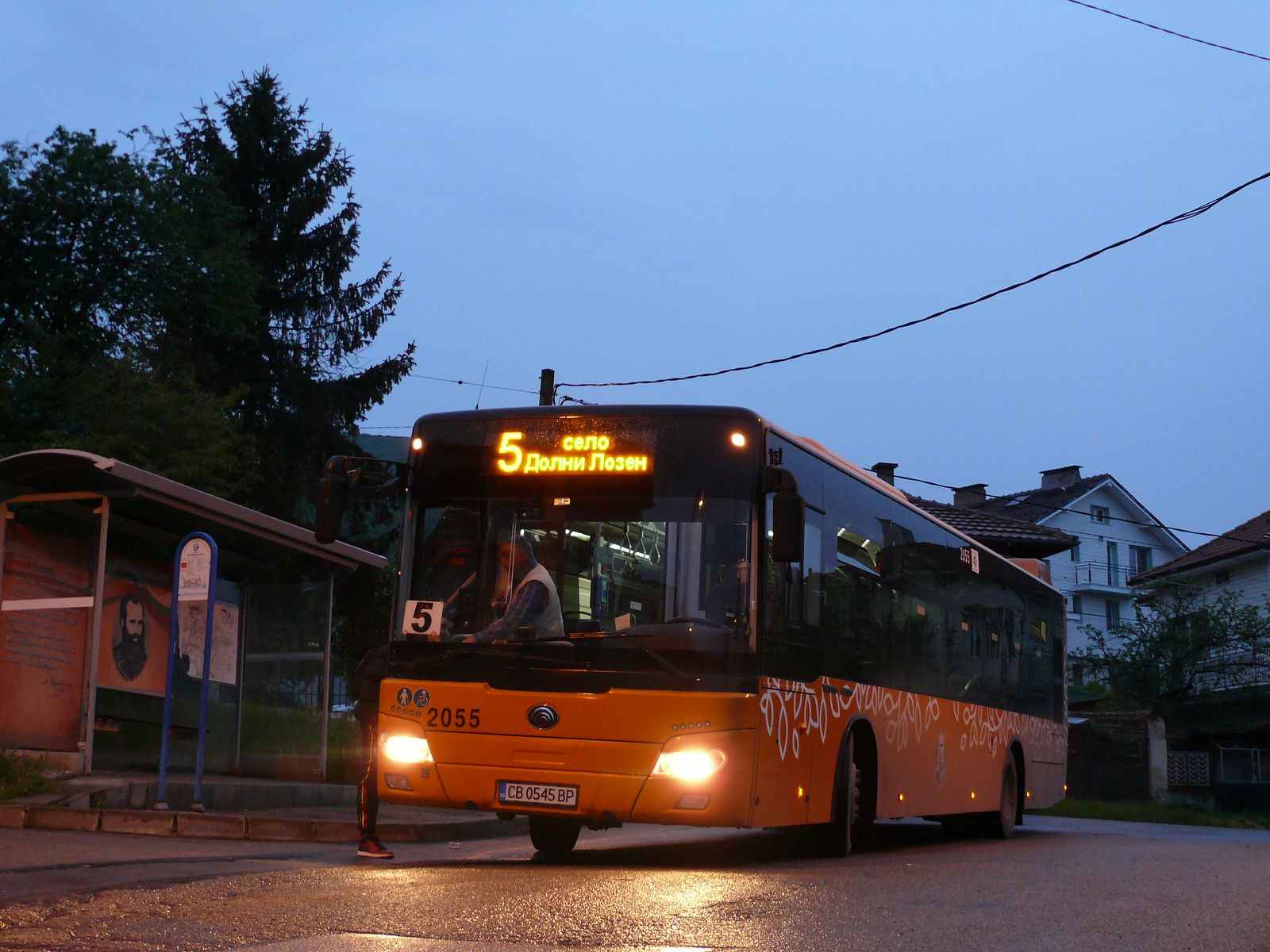The image depicts a sleek, shiny city bus, primarily orange on the lower half and black on the upper half, adorned with numerous glass windows. The orange section features a distinctive white botanical pattern, and there is some graffiti in white, though it's indecipherable. The bus, numbered 2055, has its headlights on and displays the number 5 twice—once in the front window and again on the neon destination marquee, which reads "5 Kano Borum Nossum" in what appears to be an Eastern European language. The bus stop on the left is empty, but features an advertisement with a picture of a bearded man and a blue sign shaped like an upside-down 'U'. The scene is set during twilight, with a silhouetted tree and buildings in the background, and a clear blue sky. Despite the claim that someone might be getting off, there’s no clear evidence of passengers nor any visible buses drivers in the image.